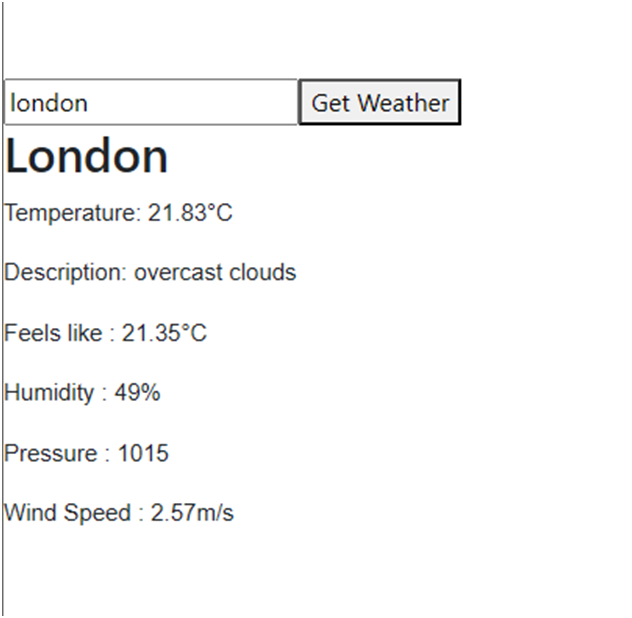This image displays detailed weather information for London, presented in a structured format. A vertical line runs down the left side of the image from top to bottom. To its right, a rectangular gray box with the word "london" in lowercase sits near the top. Adjacent to "london," there is a prompt in black text that reads "get weather."

Below this, the name "London" appears again, this time with a capital "L," in bold and larger black font. Underneath, the temperature is listed as "21.83 °C." Further details follow, including a description of the weather as "overcast clouds," with a note that it "feels like 21.35 °C." Additional information provided includes:
- Humidity: 49%
- Pressure: 1015 hPa
- Wind Speed: 2.57 m/s

The layout efficiently organizes the weather data for easy reading and quick reference.